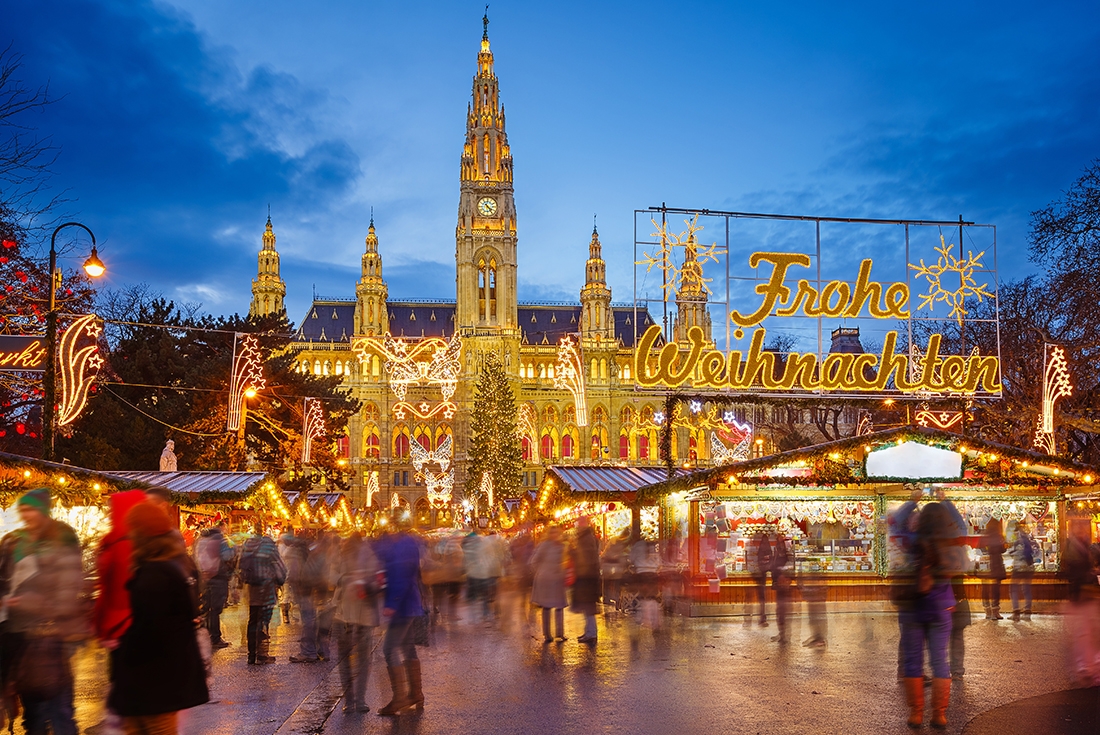The image captures a festive evening scene at a bustling Christmas market in Vienna, characterized by vibrant lights and a cold, wintry atmosphere. In the foreground, a wet ground reflects the bright illuminations, while people dressed in thick winter gear, including hats, coats, and boots, are blurred, indicating movement. These figures, though indistinct, add to the lively atmosphere as they mill about. 

Dominating the background is a majestic castle adorned in bright white lights, highlighting its architectural splendor with five spires—two lower spires on each side and a tall central clock spire. The castle features numerous windows and archways, enhancing its grandeur. Centrally located in front of the castle is a Christmas tree, also draped in white lights, that reaches halfway up to the clock spire, stopping just below the windows. 

To the right of the photo, partially obscured, is the end of the word "market" in Vienna's language, brightly lit with yellow or white lights accompanied by stars. On the left side, a lit-up sign spells "Frohe Weihnachten" in large cursive letters, with "Frohe" on the top line, flanked by snowflakes, and “Weihnachten” below. This sign is situated above one of the market stands, which is illuminated by a bright white light. The temporary structures of the stands blend into the festive atmosphere though details of the signage are blurred.

Overall, the dark blue sky with gray clouds enhances the evening ambiance, emphasizing the warmth and brightness of the Christmas lights, creating a picturesque holiday setting.